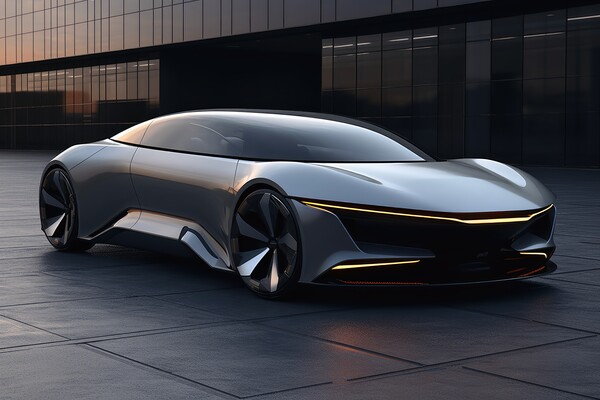This is a color photograph of an incredibly sleek and futuristic-looking sports car. The car, which has a modern and aerodynamic design, is a striking slate gray or charcoal gray color, and features a highly reflective, chrome-like finish that glistens as the light reflects off the paint. The photograph captures the car from an angled perspective, showing the passenger's side and oriented towards the bottom right. The car's most distinctive design element is its seamless glass top, which extends from the front all the way to the back. This gives it a very sleek appearance, with no visible doorknobs—it’s all smooth, possibly suggesting that the doors may open in an unconventional manner, perhaps from the roof.

The tires are notable for being almost as tall as the entire height of the car, suggesting high-performance capability. The front of the car resembles that of a Tesla, with flat surfaces and highlighted by a bright yellow striping across the front, adding a touch of vibrancy to its modern design.

The car is parked on a gray, tiled paver surface that resembles charcoal gray in color. It is set against a backdrop of a very modern building with dark, glass windows. The sun is setting, casting a warm reflection onto the building, which further enhances the sleek and futuristic ambiance of the scene.